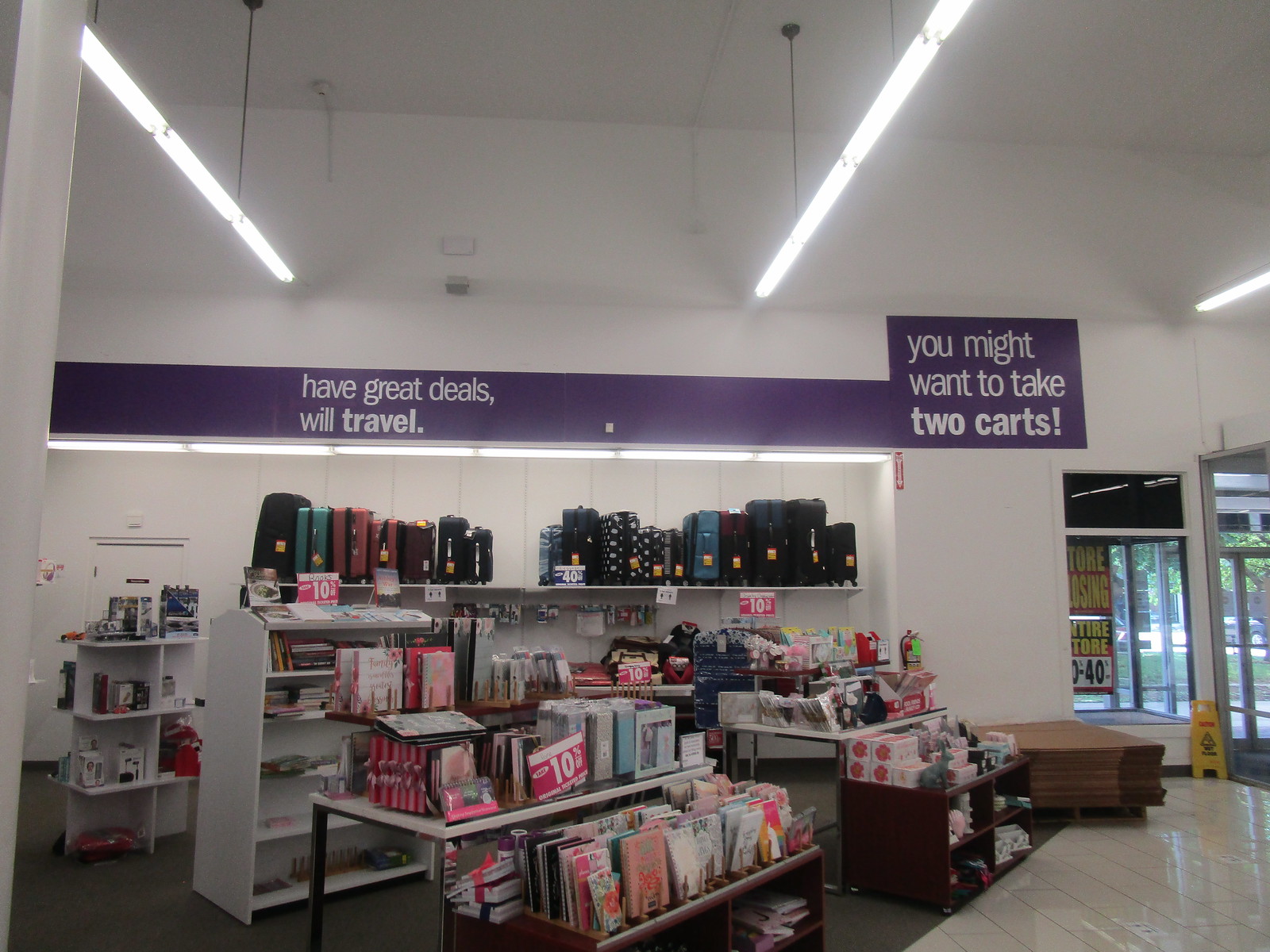This photograph captures the interior of an outlet store characterized by its prominent white walls and bright, vertically-hung fluorescent lights attached to the ceiling. A significant feature is a large purple banner with white text reading "Have great deals, will travel. You might want to take two carts," positioned high on the wall. Below the banner, there are several shelves filled with suitcases of various shapes and colors arranged in neat rows. Closer to the foreground, additional shelves are stocked with assorted supplies, including journals. On the right side of the image, the store's entrance is visible, adorned with a window banner indicating the store is closing, offering discounts ranging from an unspecified amount up to 40%. Near the entrance is a yellow fold-out caution sign warning of a wet floor. The store's floor combines gray carpet on one side and white tile on the other, adding to the organized layout of the retail space.